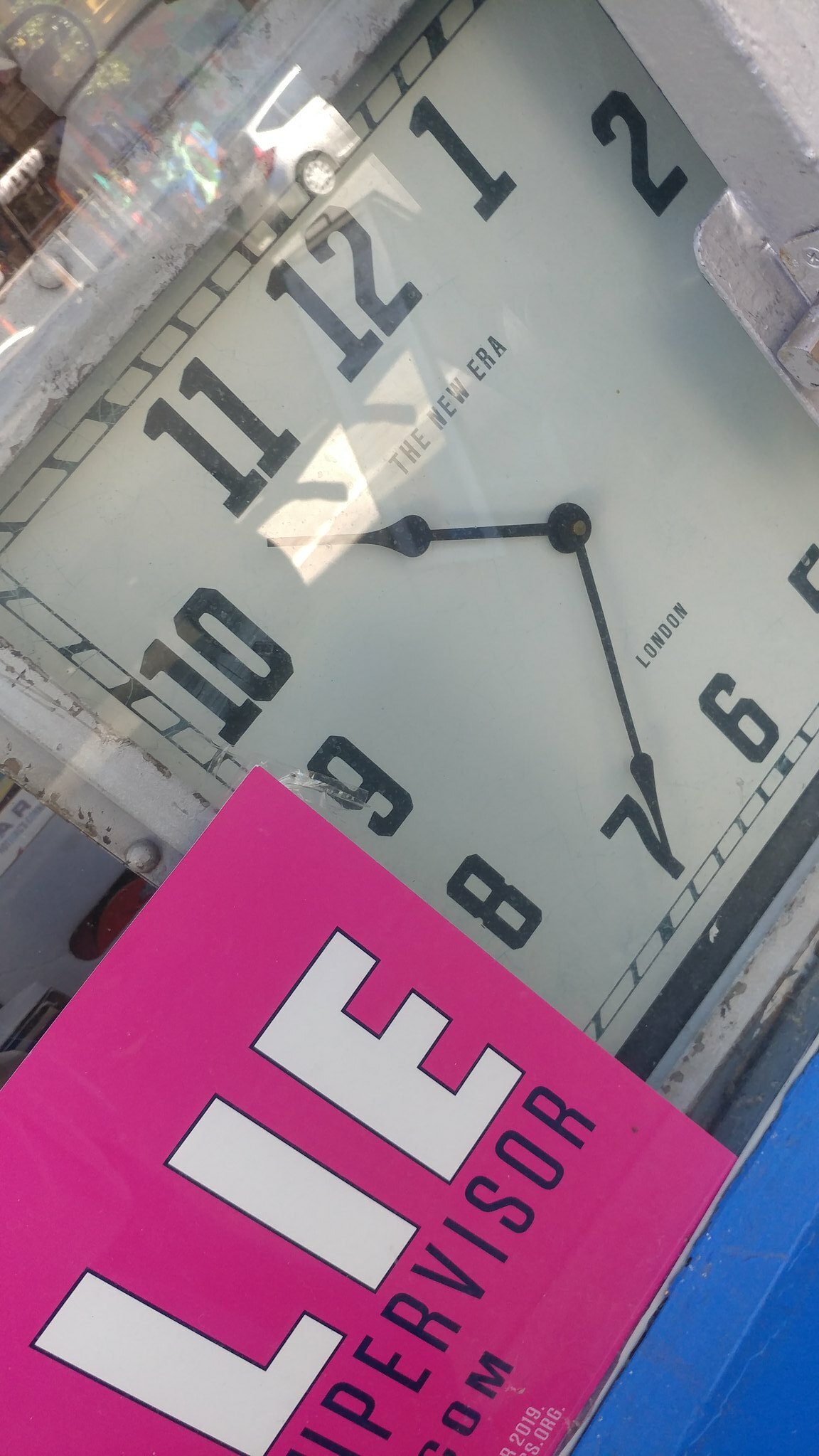A close-up photo displays a square clock for sale, possibly encased in a glass cabinet given the noticeable reflections and a faint outline resembling a cabinet door mechanism in the upper right corner. The image is tilted, with the top of the clock, including the '12,' tilted left, positioning it between the '1' and '2.' A triangle of blue occupies the lower right corner, while the left corner reveals a section of a sign on a dark pink background, reading "L-I-E" in white letters. Below, partially obscured, are the words "supervisor" and possibly "C-O-M." The clock, bearing the text "The New Era" along with "London" above the '6,' indicates the time as 10:35. Signs of wear, such as rubbed and dirty edges, suggest that the clock may not be brand new.